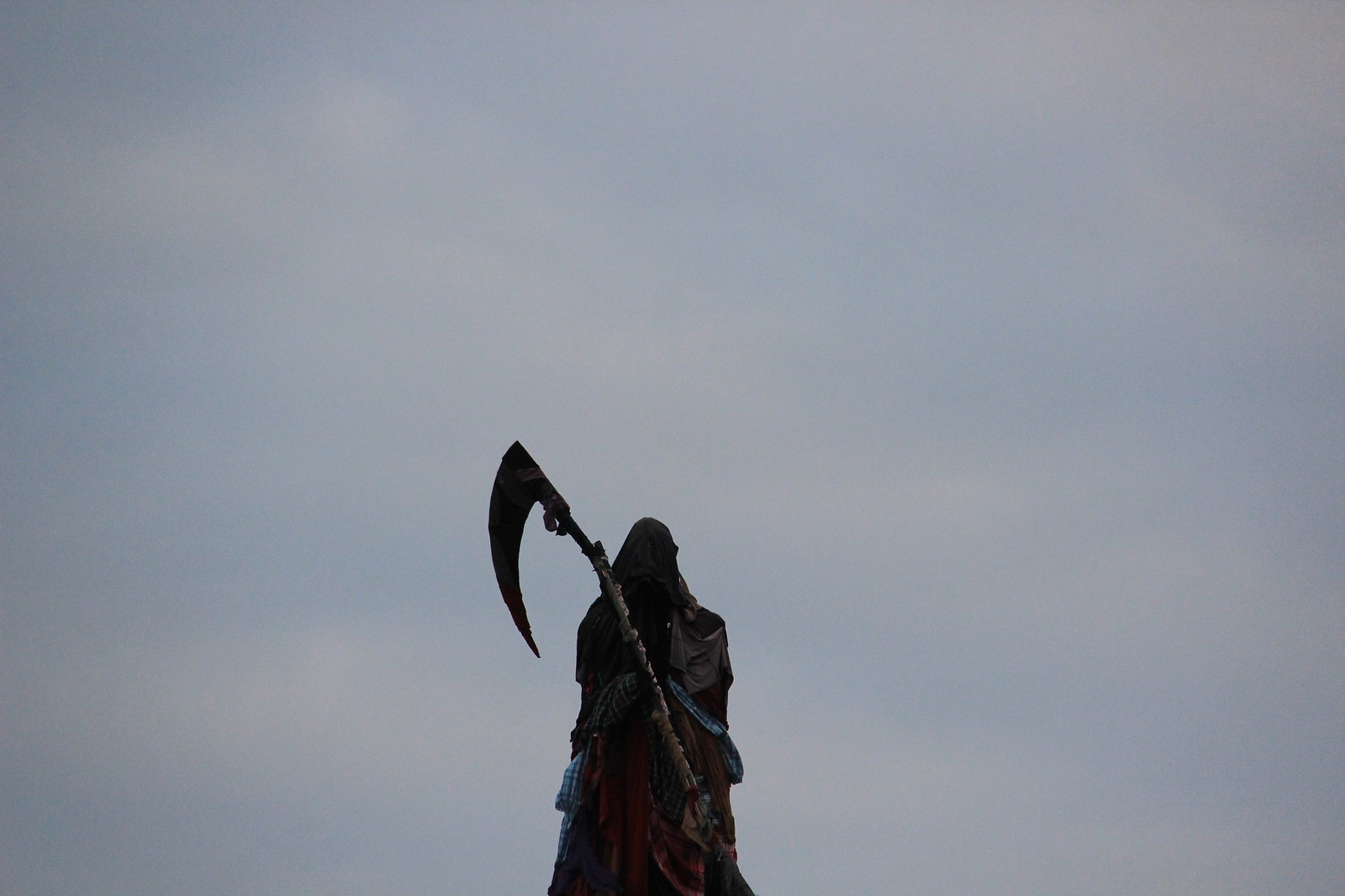The image portrays a striking statue of the Grim Reaper, centrally positioned in the frame. The ominous figure is cloaked in a variety of draping materials in numerous colors—reds, blues, and greens—with the hood and facial area predominantly shrouded in black and gray. The statue, possibly crafted from bronze or metal, stands with a menacing scythe poised over its shoulder, the curved blade extending three to four feet. The sculpture's detailed folds and contours are accentuated against the backdrop of a cloudy, overcast sky, tinged with hints of blue and white mist, suggesting either an outdoor setting or an ambiguous indoor background. The atmospheric lighting hints at a possible twilight scene, adding to the eerie and dramatic effect of the Reaper's presence.